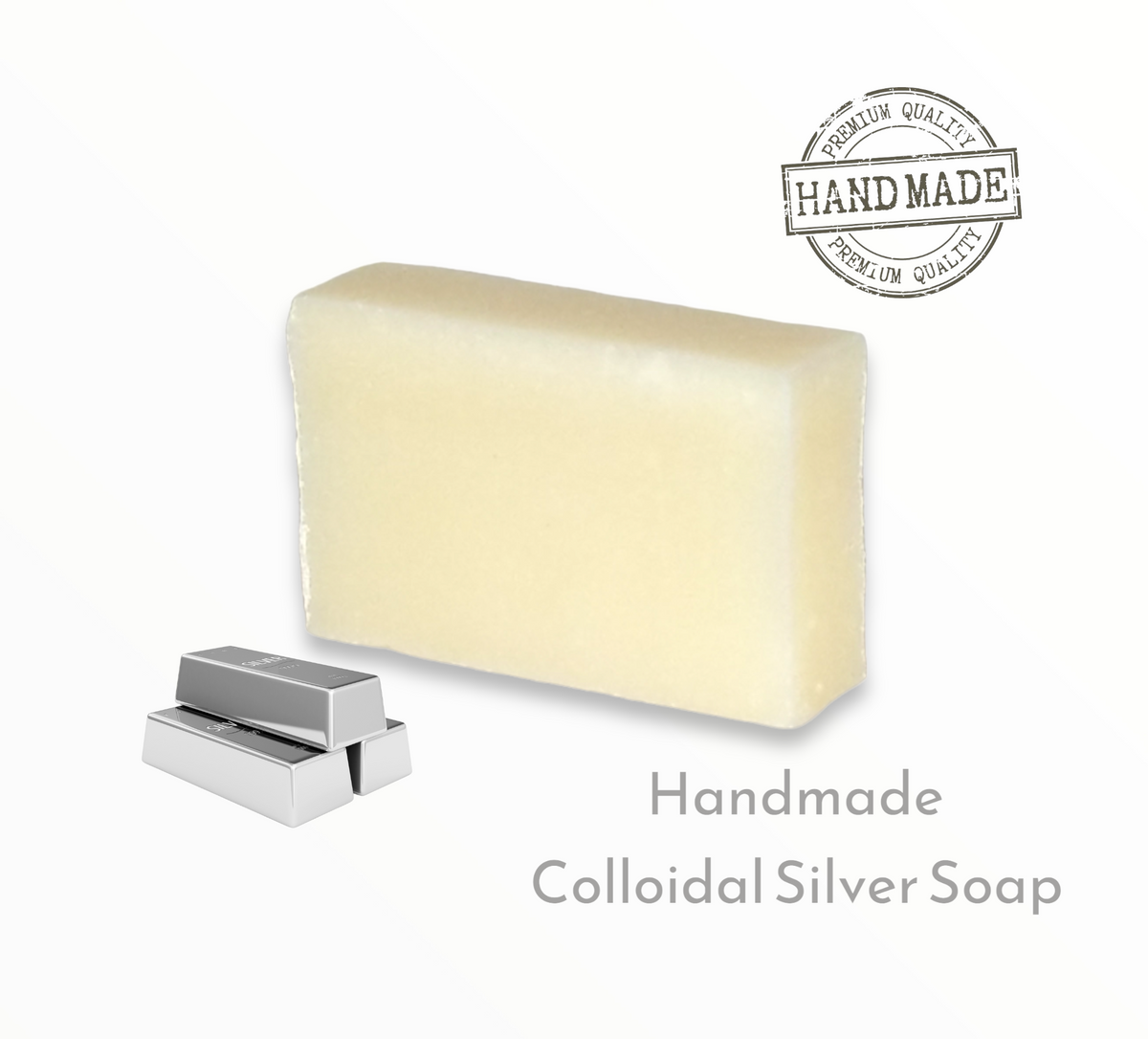The photograph showcases a white, rectangular bar of soap positioned against a white background, giving it the illusion of floating in a void. The soap is angled, revealing its front and right side while obscuring the left. At the top right corner of the soap is a graphic seal reading "Premium Quality, Handmade, Premium Quality." On the bottom left, there are three stacked bars of silver metal. Adjacent to these bars, in gray text, is the inscription "Handmade Colloidal Silver Soap," strongly suggesting the use of silver in its handcrafted production process. The predominant colors in the image are cream, silver, black, and brown, contributing to a clean and premium aesthetic.